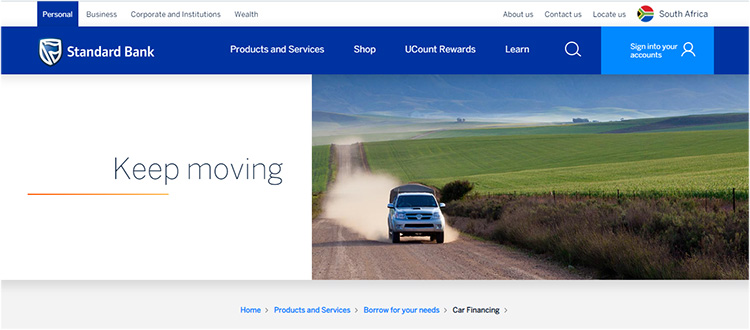On this webpage from Standard Bank, the header features several navigation tabs: "Personal," "Business," "Corporate Institution," and "Wealth." The "Personal" tab is highlighted in blue on the left side, signifying the selected section. In the top right corner, there are additional links including "About Us," "Contact Us," "Locate Us," and "South Africa." Adjacent to the "South Africa" link is a flag of South Africa with six colors: red, green, black, yellow, white, and blue.

Beneath the main tabs, the Standard Bank logo and name are prominently displayed. The lower header area has more tabs including "Products and Services," "Shop," "Your Account Rewards," and "Lend," along with a search icon. The background here is a dark blue color, and a "Sign In to Your Account" button, also in blue, is located to the right.

On the right side of the page, there is a banner with the text "Keep Moving" in black against a white background. An orange line runs below this text. Below the banner, a silver-grey car is depicted driving on a gravel road towards the right side, leaving a trail of dust. The surroundings include green fields on both sides of the road.

At the footer of the page, there are several navigation buttons: "Home," "Products and Services," "Borrow Your Needs," and "Car Financing." All buttons are blue except for "Car Financing," which is written in black, indicating it is selected or highlighted.